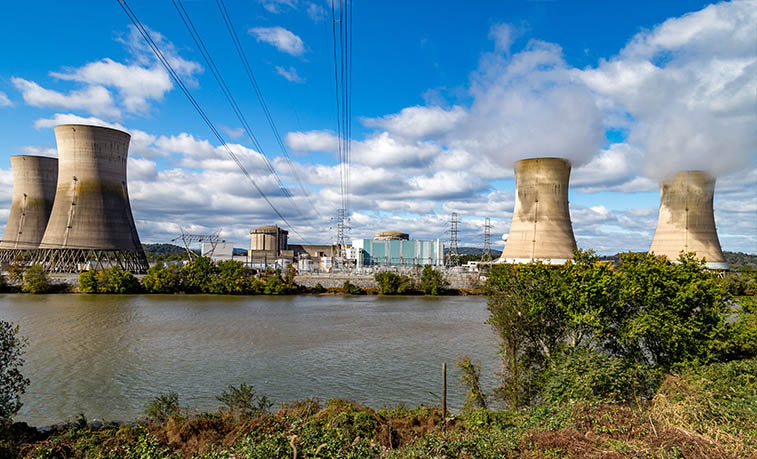The photograph captures a detailed view of a nuclear power plant set against a backdrop of a brilliant blue sky adorned with puffy white clouds. The power plant is characterized by four distinctive cooling towers arranged from left to right, with the two on the right actively emitting steam or vapor, indicating they are in operation. The cooling towers have the familiar sloped cylindrical shape, and the structure of the plant includes two visible reactor domes along with several other buildings. Situated behind a large reservoir, the scene also features a mix of shrubby greenery around the water's edge. Power lines and transformer wires are seen running from behind the camera towards the power station. The concrete structures, with their grayish-yellowish hue, stand in stark contrast to the vibrant natural elements and the azure sky, creating a visually striking composition.